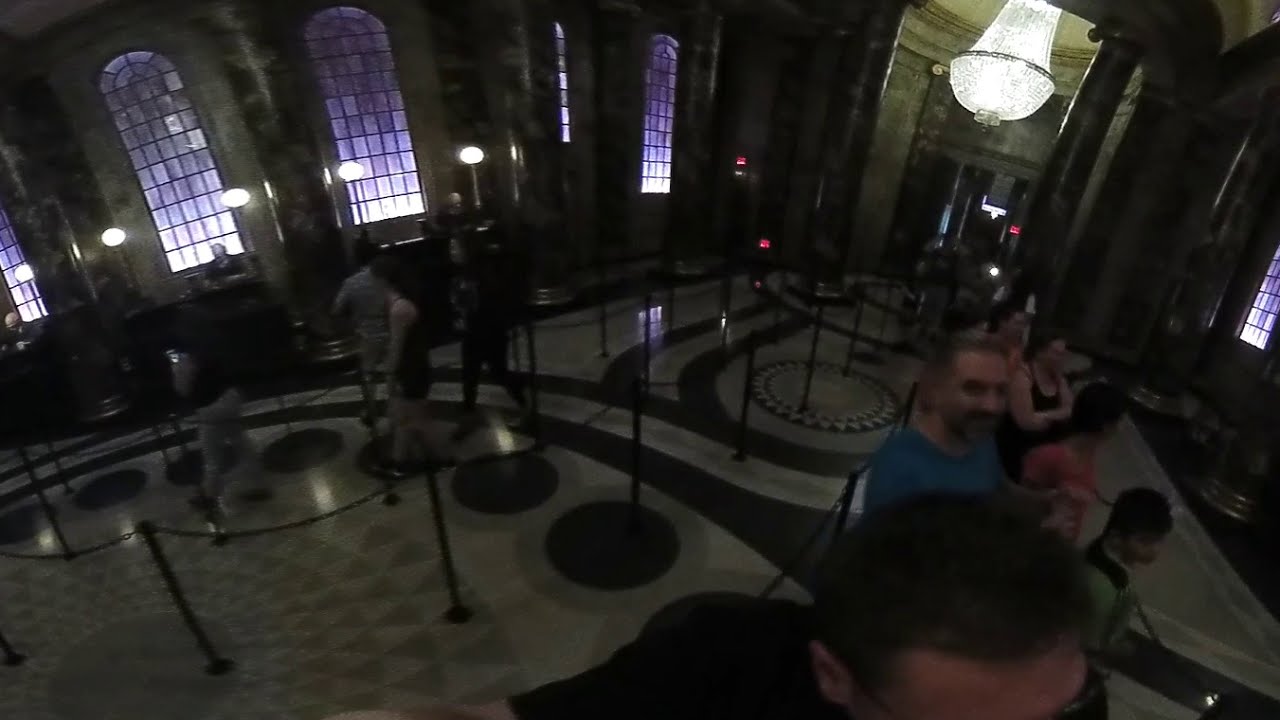This photograph captures the ornately intricate interior of an expansive, historical museum, possibly a former governmental building based on its grand architecture. The room is characterized by its high, arched ceiling supported by large marble columns, creating an atmosphere of both grandeur and solemnity. Despite the richness of the architecture, the lighting is relatively dim, with only a few bright spots such as the massive, luxuriant chandelier towards the top right of the image, emitting a soft yellow light that accentuates its crystalline structure.

The floor features an elaborate starburst design, indicative of the careful craftsmanship that went into constructing this edifice. The overall color palette is muted, with shades of brown and tan dominating the scene. The tall, arched windows—tinted in hues of blue, purple, and white—allow diffused light to filter into the space, adding to the ethereal quality of the room.

A significant number of visitors are present, possibly tourists or museum-goers, forming long lines along roped-off queues. These lines suggest they are waiting to view various exhibits or perhaps proceeding towards a counter area situated in the background. The demographic includes both adults and children, indicating the site’s broad appeal. Despite the crowd, there's a sense of orderly progression among the visitors, adding to the scene's structured yet bustling atmosphere.